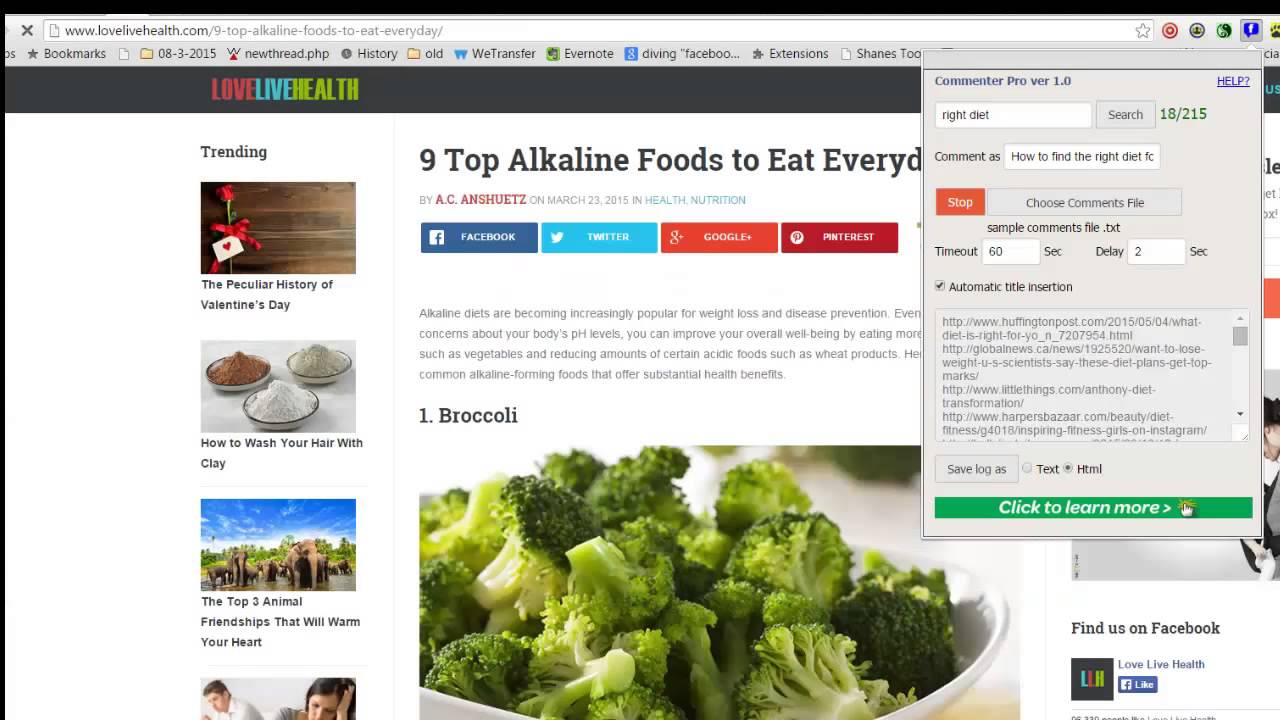This is a screenshot from the website www.lovelivehealth.com. The central focus of the screen is a blog article titled "9 Top Alkaline Foods to Eat Every Day." The article is accompanied by an image of a bowl filled with cooked broccoli placed in a white bowl. In the upper right-hand corner of the screen, there is a pop-up window displaying information about the current version of the app being used. On the left-hand sidebar, there are thumbnails and titles of trending articles. The top trending article delves into "The Particular History of Valentine's Day," followed by an article on "How to Wash Your Hair with Clay," and another on the "Top Three Animal Friendships That Will Warm Your Heart."